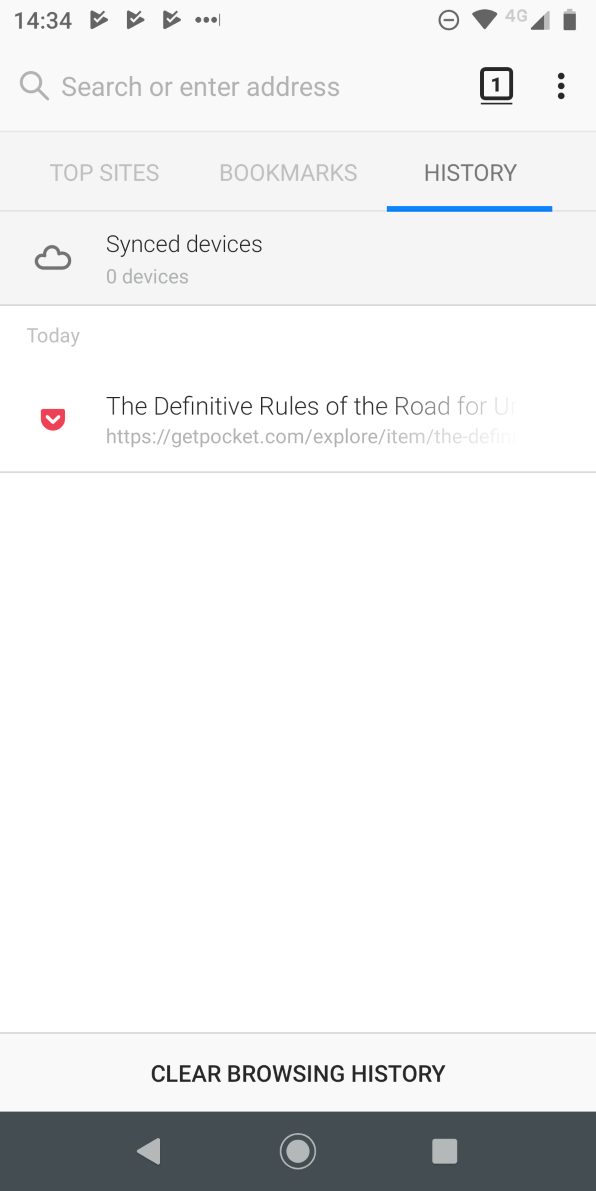The image shows a screenshot of a cellphone screen with detailed elements spanning from the top to the bottom. In the top left corner, the time is displayed as 14:34. Adjacent to this, there are three triangles, each marked with check marks. On the right side of the screen, there are three vertically aligned dots. Next to these, a "Do Not Disturb" symbol is present, alongside icons for Wi-Fi, 4G signal strength, and battery status.

Below the status bar, there is a search bar reading "search or enter address," accompanied by a search icon. Nearby, there is a box with the number "1" inside it, followed by three vertical dots. Beneath this section, there is a light gray line with the words "Top Sites," "Bookmarks," and "History" arranged in a row. The "History" tab has a blue underline, indicating it is the active section.

Further down, there is a section labeled "Sync Devices (0 devices)." Under a heading marked "Today," there is a partially visible text headline, "The definitive rules of the road for," which appears to be truncated. The source link "https://getpocket.com/explore/item/the-" fades out as well. Another gray line separates this text from a large white space, followed by another gray line with the text “Clear Browsing History” prominently displayed in black capital letters.

The bottom of the screen features a black navigation strip with three icons: a left arrow, a circle, and a square, depicting the cellphone’s navigation buttons. The color scheme predominantly consists of black, gray, blue, red, and white, with several shades of gray.